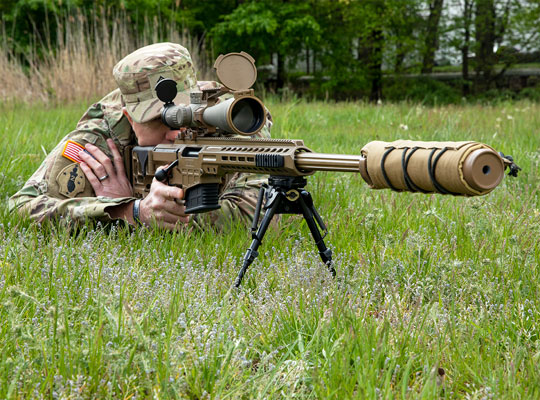In this detailed outdoor daytime photograph, a middle-aged Caucasian soldier, likely a sniper, is seen lying prone in a grassy field adorned with tall dried grass, various weeds, and small purple flowers. The soldier is clad head-to-toe in camouflage gear, including a hat and a uniform featuring an American flag patch on the sleeve. On the soldier's left hand, a silver wedding ring and a metal bracelet are visible. Positioned on a tripod in front of the soldier is a large khaki-colored gun, its barrel wrapped in what appears to be burlap for noise reduction. The soldier's focused gaze is locked through the gun's substantial scope, their finger poised on the trigger. Behind them, a serene forest frames the scene, while a car-free road is also discernible in the distant background. The atmosphere conveyed suggests the dedicated precision and readiness typical of a sniper in their element.